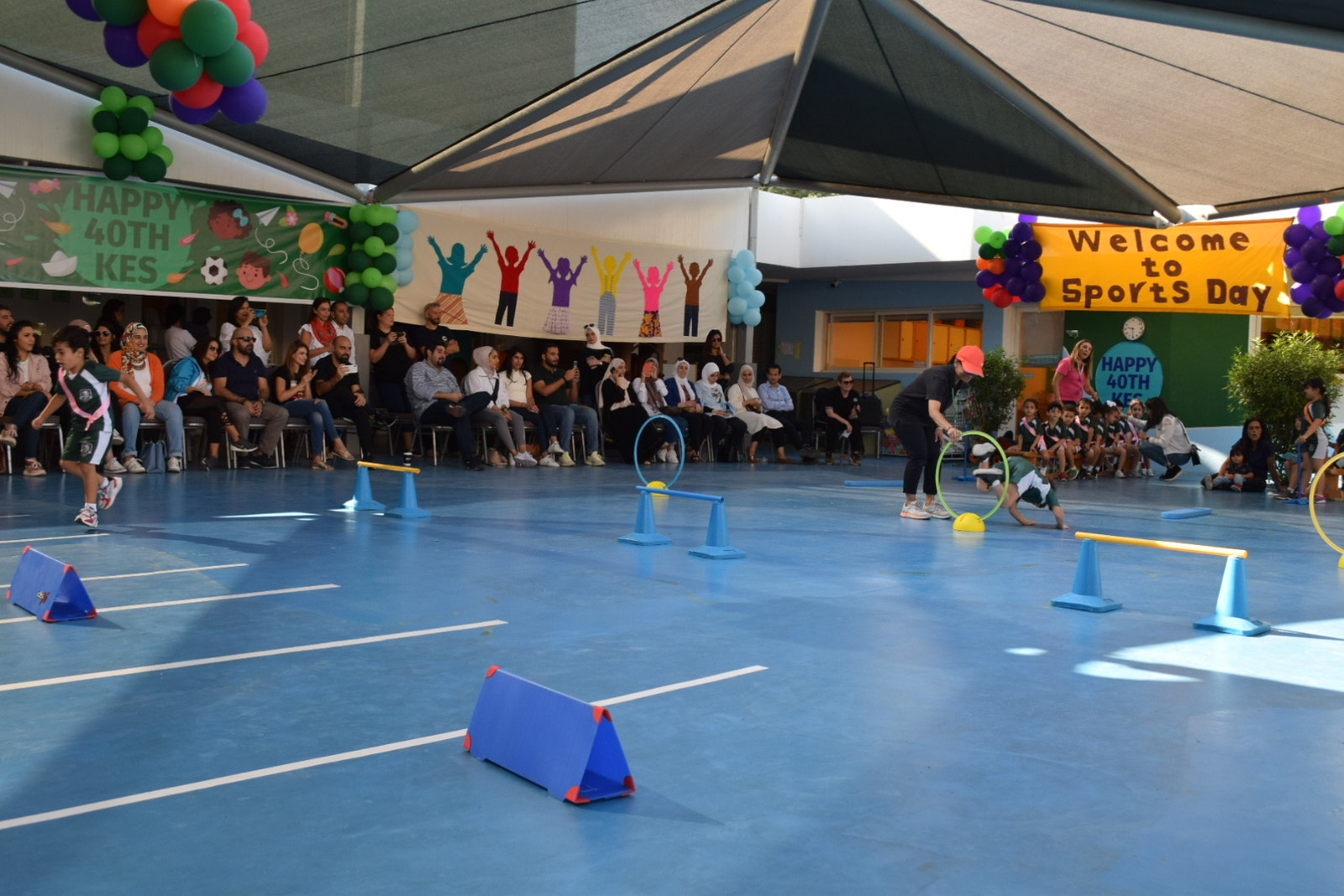The image depicts an outdoor event in a blue-floored courtyard, possibly part of a school's celebration. The scene is covered by a tent that peaks in the middle, giving shelter to the activities below. Prominently displayed on the left wall are murals, one green and one white, both featuring colorful silhouettes, along with a message reading “Happy 40th KES.” A matching banner on the right reads “Welcome to Sports Day.” Spectators, including parents and children, are seated on the left side, watching the lively scene. The event appears to include an obstacle course with various setups such as hurdles and hula hoops on pedestals. In the center left, a young boy dressed in navy sportswear runs toward the left side, while nearby, a woman in an orange cap bends over a yellow hoop, preparing for a small dog to jump through. The photograph captures the essence of a festive, community-oriented sports day, celebrating the 40th anniversary of KES, with balloons in blue, orange, and green adding to the cheerful atmosphere.